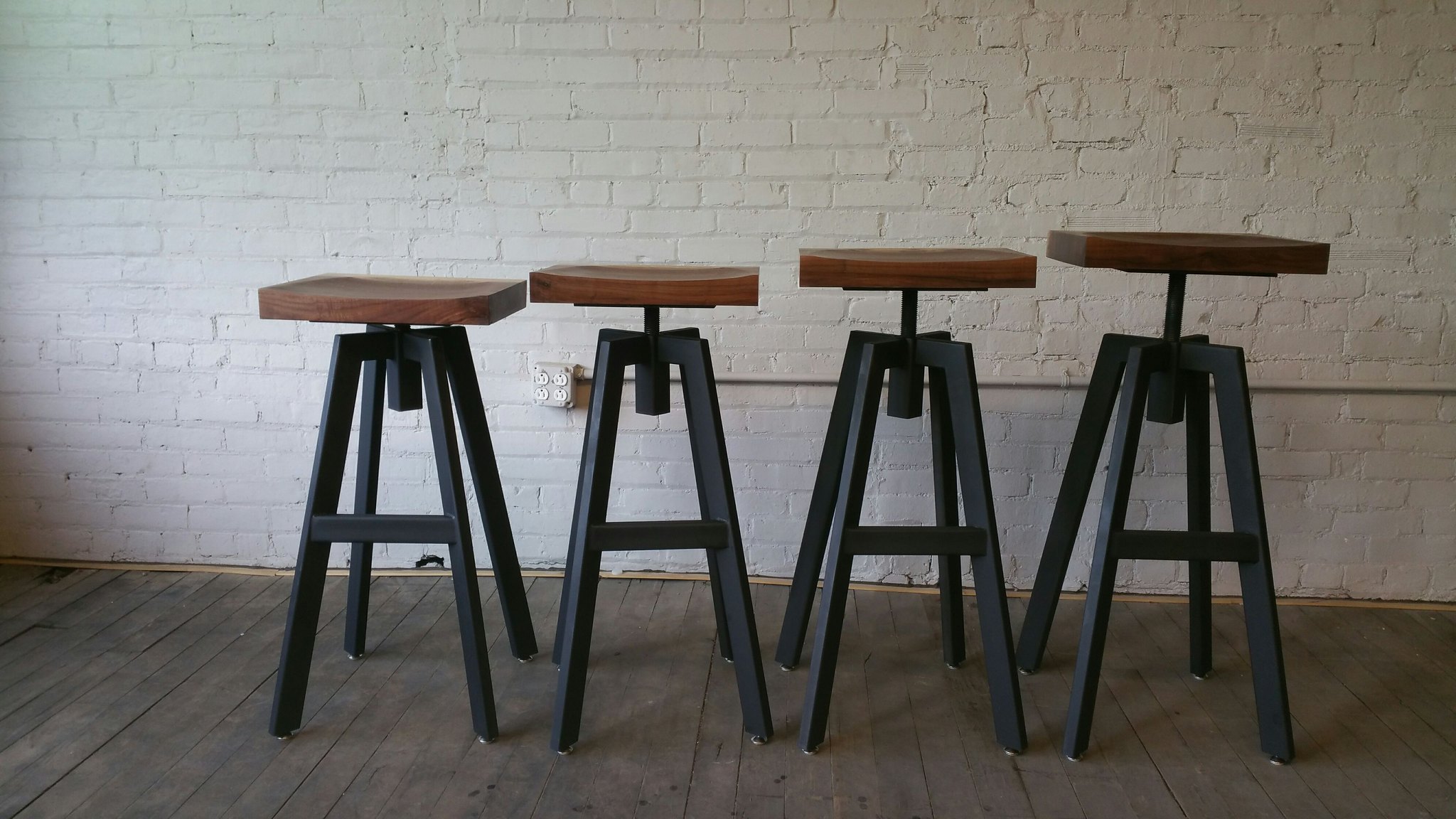The photograph showcases a series of four backless barstools arranged from left to right on a distressed, narrow wooden hardwood floor. Each stool features a dark brown wooden seat supported by a matte black base with four legs that slightly splay outward, equipped with silver attachments at the bottom for stability. The stools progressively increase in height from left to right and appear adjustable, indicated by mechanisms beneath the seats. A horizontal bar provides extra support between the front and back legs of each stool. The background consists of a white-painted brick wall, which has visible light sources casting shadows and includes a power outlet and an electrical pipe running across its surface.